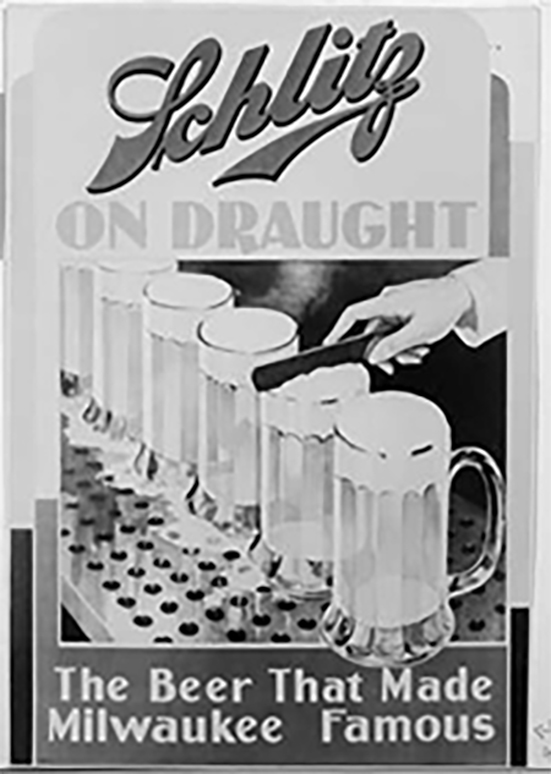This poster from the 1940s or 1950s advertises Schlitz beer with the slogan "The beer that made Milwaukee famous." At the top, in a diagonal cursive script reminiscent of baseball jersey fonts, the word "Schlitz" is featured prominently. The "z" in Schlitz creates a distinctive line under the other letters. Below this, in a lighter color, it reads "On Draught." The image shows six glass beer mugs, filled to the brim and neatly aligned diagonally from the lower right to the upper left corner, atop a metal surface dotted with small holes, functioning as a drain. A hand in a light-colored t-shirt is visible on the right, using a flat, knife-like tool to scrape the foam off the tops of the beers. The scene is rendered in a mostly black and white palette, and the entire composition is framed within a tall rectangular shape.